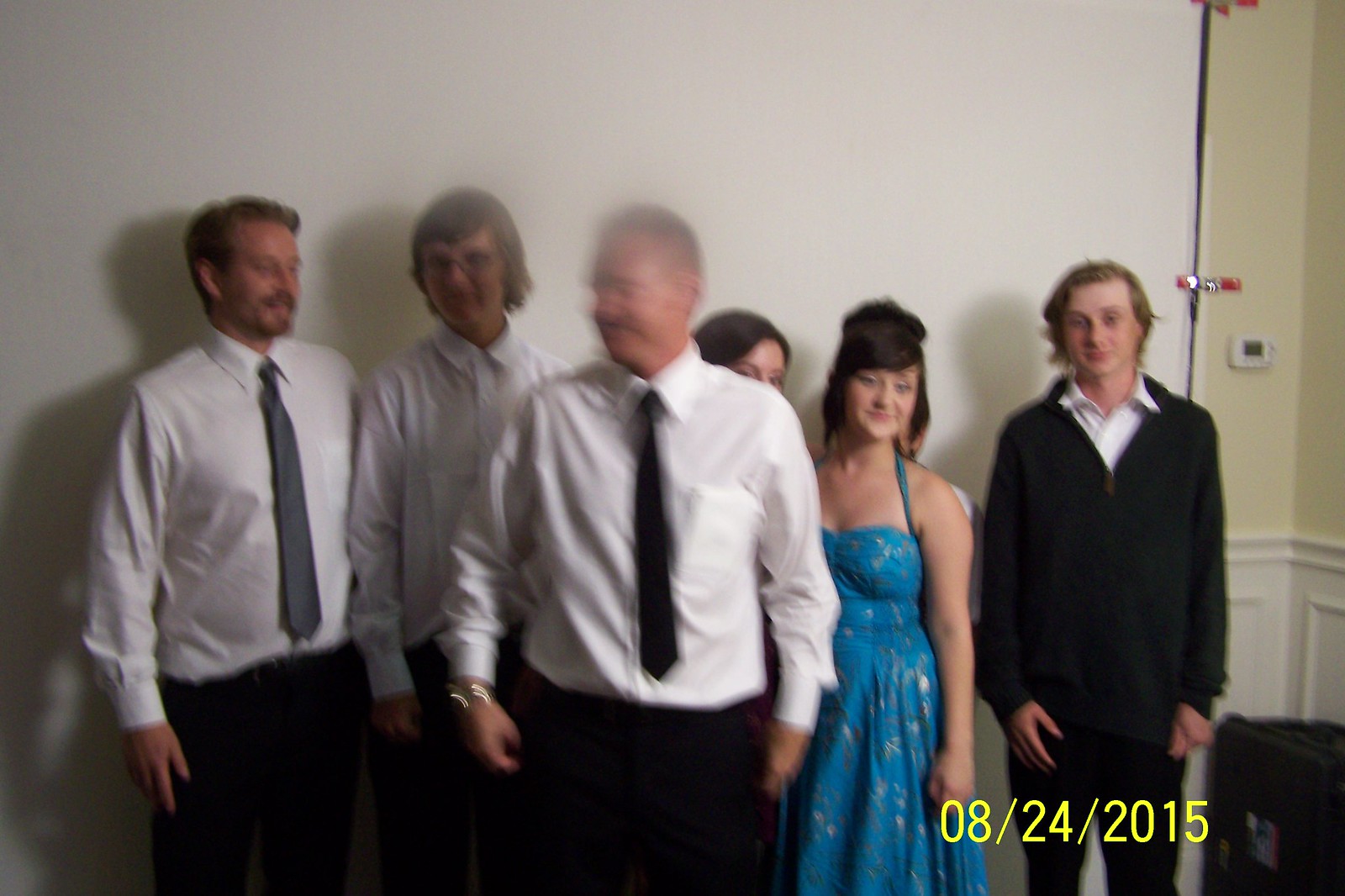The image, dated 08-24-2015 in yellow font at the bottom corner, captures a moment indoors within a spacious room. Despite its slight blurriness, the photo features six individuals. At the forefront, there are three men, each clad in white long-sleeve button-up shirts and black pants. Two of them are wearing ties—one in black and the other in gray—while the man in the middle does not have a tie. Behind them, a female figure is partially visible, with only her eyebrows and the top of her head discernible. To their side, a teenage girl, her hair elegantly styled up, stands out in a prom dress. Accompanying her is a young man. The setting conveys a blend of formality and youthful celebration.